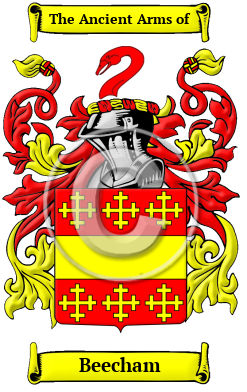This detailed illustration features the ancient arms of Beecham. The image prominently showcases a family crest with a yellow scroll at the top bearing the words "The Ancient Arms," and another yellow scroll at the bottom with the name "Beecham" inscribed in black letters.

The central element of the crest is a shield that sports red and gold (or yellow) colors adorned with intricate cross symbols arranged within crosses, which evoke a medieval aesthetic. Rising from the top of the shield is a traditionally styled knight's helmet, depicted with a visor pulled down, signifying the warrior lineage of the family.

Emerging from the helmet is a distinctive figure that appears to be a red bird, possibly a stylized goose or another avian creature, adding a unique and striking element to the crest. Flanking the helmet and the bird are elaborate, flowing vines resembling leafy tendrils, enhancing the heraldic grandeur of the image. Surrounding the head, additional decorative elements include leaves and draping cloth, contributing to the ornate and historical feel of the Beecham coat of arms.